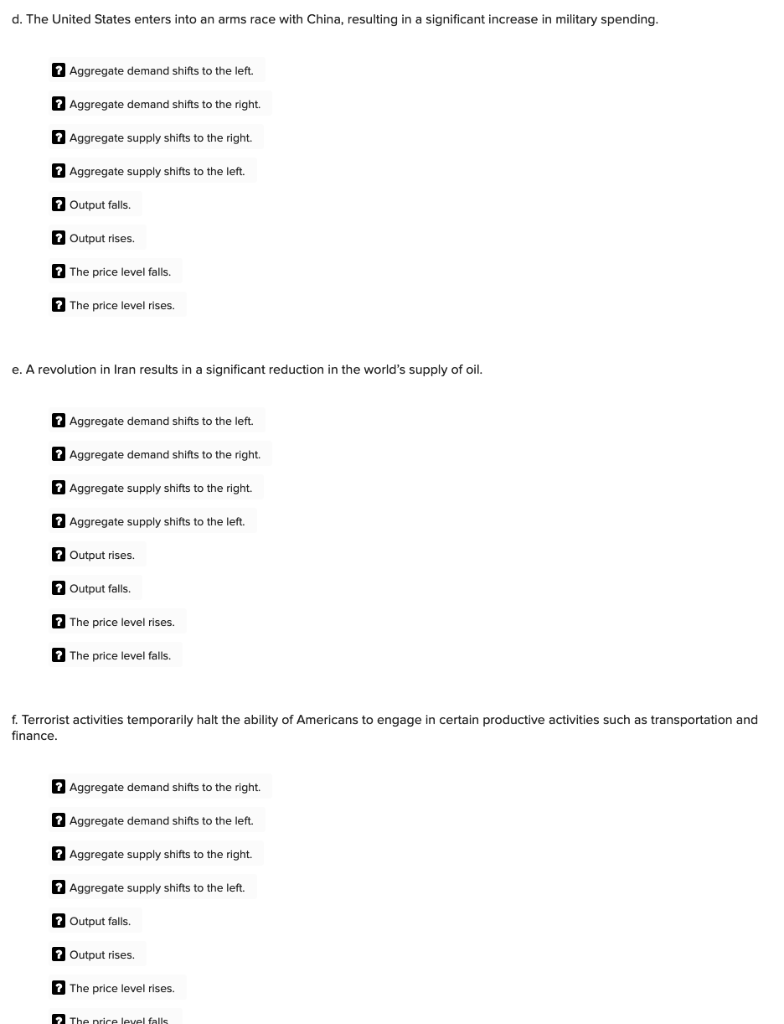The image is a text-laden graphic, primarily in black text on a white background, detailing various economic scenarios and their potential impacts on aggregate demand, aggregate supply, output levels, and price levels. Here is a refined and descriptive caption:

---

**Detailed Analysis of Economic Scenarios and Their Impacts on Aggregate Metrics**

The image comprises a comprehensive list of economic scenarios, each followed by a series of potential outcomes for aggregate demand (AD), aggregate supply (AS), output, and price levels. The scenarios listed include:

1. **China's Increased Military Spending**: This scenario results in multiple possible shifts in economic aggregates – aggregate demand shifts to the left or right, aggregate supply shifts to the right or left, output falls or rises, and the price level falls or rises. Each possibility is marked with question marks, indicating selectable options.

2. **Revolution in Iran**: This event leads to a considerable reduction in the world's oil supply. The image lists potential economic responses, including shifts in aggregate demand to the left or right, shifts in aggregate supply to the right or left, changes in output (rising or falling), and fluctuations in the price level (rising or falling). Again, each outcome is denoted with a question mark indicating options.

3. **Terrorist Activities Affecting U.S. Productivity**: The scenario where terrorist activities temporarily disrupt American productivity in sectors such as transportation and finance is presented. The potential economic impacts are detailed similarly, with options for aggregate demand shifting left or right, aggregate supply shifting left or right, changes in output levels, and varying price levels.

The entire image focuses solely on presenting these textual scenarios and their possible economic implications, arranged methodically for ease of understanding and analysis.